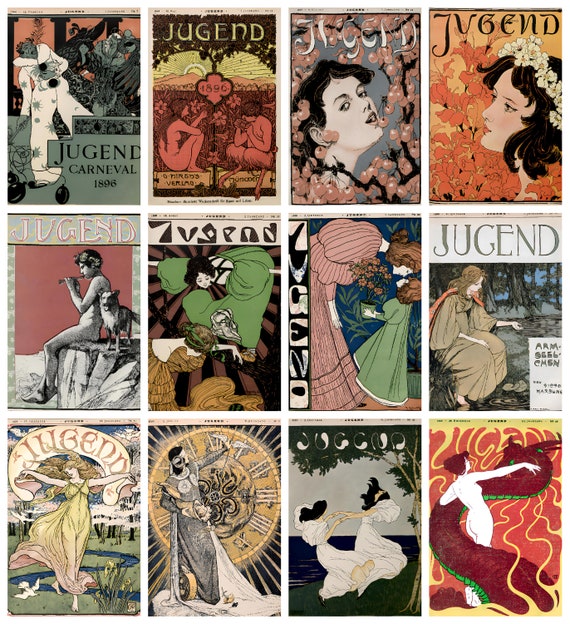This image showcases a collection of twelve Jugend magazine covers from the late 1800s to early 1900s, arranged in three rows of four. The covers are unified by the magazine's title, "Jugend," prominently displayed in the distinctive, swirling letters characteristic of the Art Nouveau style. The collection features various themes and vibrant illustrations, with a notable emphasis on colorful depictions of women. One cover, dating to 1896, specifically highlights a "Jugend Carnival" and features a whimsical clown figure against a predominantly green backdrop. Another striking cover from the collection portrays a woman adorned with a floral headband, gazing upwards to the left with orange flowers serving as the background. Among the assortment is also a cover depicting two women in white, dancing gracefully. The themes of the artwork vary widely, with some covers incorporating Asian-inspired elements such as Geisha figures, and others suggesting influences from French, Greek, and Roman aesthetics, as well as depicting mythical creatures like dragons.